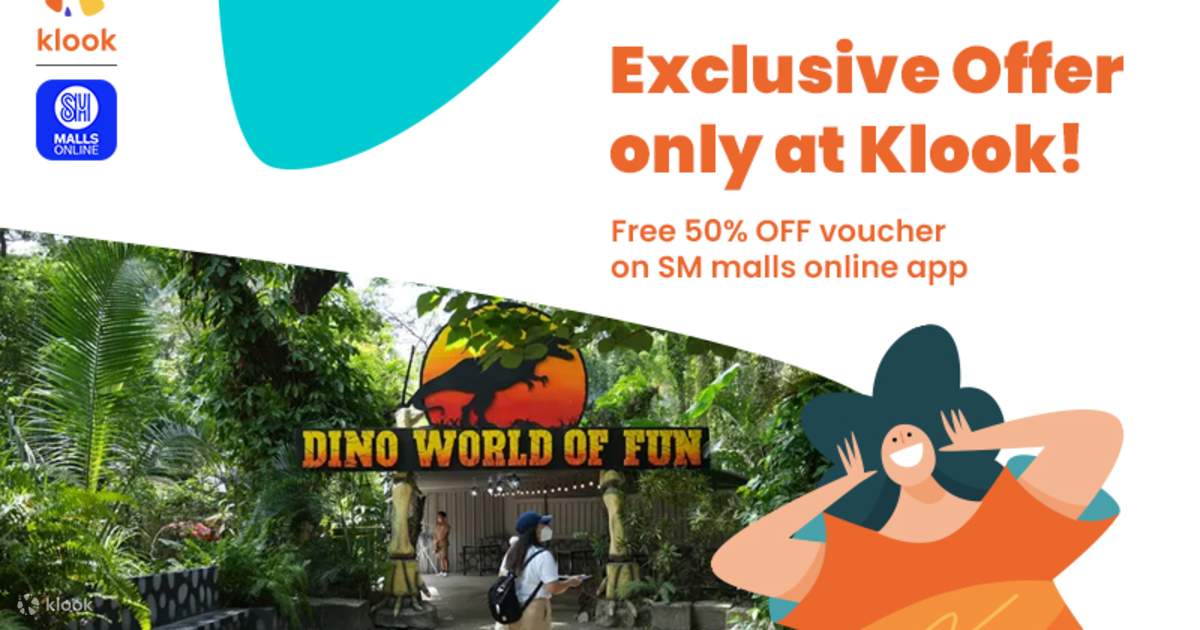The image showcases a promotional banner for Klook, highlighted by its logo in the upper left corner, followed by the "MallsOnline" branding in white font set against a blue background. A large, eye-catching turquoise blip descends from this section. To the right, the banner announces in bold orange text, "Exclusive offer only at Klook: Free 50% off voucher on SM MallsOnline app." 

At the bottom right of the image, a cartoon woman is depicted with her hands cupped around her mouth as if yelling. She wears an orange T-shirt with a turquoise-blue inner design, complemented by her large black hair and peachy-brown skin tone. Her open mouth, revealing a white interior, and her black-dot eyes suggest excitement. 

Adjacent to the cartoon woman is an image with the text "Dino World of Fun" set against a backdrop reminiscent of a photograph from an amusement park, which bears a visual similarity to the iconic "Jurassic Park" sign. The logo reads "Dino World" in striking yellow on the top and orange on the bottom, all set against a black background teeming with real-life visitors and vivid green plant life. 

The text and other design elements are laid on a white backdrop, with the amusement park photo curving out from the left side and creatively blending behind the cartoon woman on the right. This composition balances between stark whites and lush greenery to emphasize the vibrancy and allure of the promotional content.